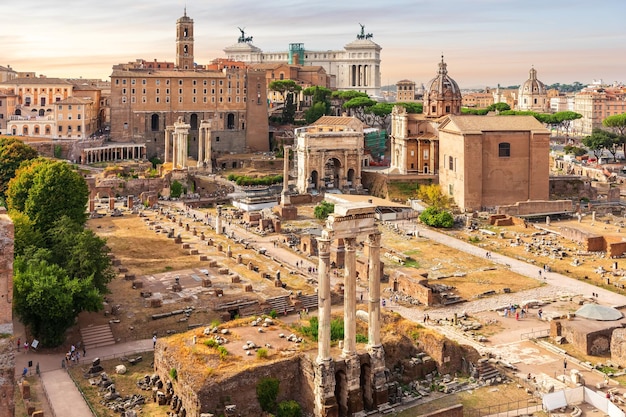The image depicts an expansive aerial view of an ancient city marked by ruins and partially preserved structures. Dominating the foreground is a raised platform adorned with three tall, roofless columns standing amidst broken rock. The scene transitions into a grid-like road and a large rectangular flatland featuring rows of stubby cylindrical remnants, hinting at the foundations of long-lost buildings. To the right, another similar flat expanse can be seen.

Midway through the image, a thoroughfare bordered by sand-colored and white buildings, some up to five stories high, meanders towards the background. Among these structures, a prominent tower and an array of arches, including a wall with three distinct archways, are notable. Further back, dense rows of trees provide a verdant frame to this historical tableau.

The distant horizon showcases diverse architecture, with several arches and two domed buildings punctuating the skyline. All of this is bathed in the warm, amber glow of a setting sun, its light casting an ethereal hue across the clear, light blue sky adorned with a hint of orange. Scattered throughout the cityscape, tourists wander among the ruins, capturing glimpses of the past on what is evidently a sunny day ideal for exploring this storied site.